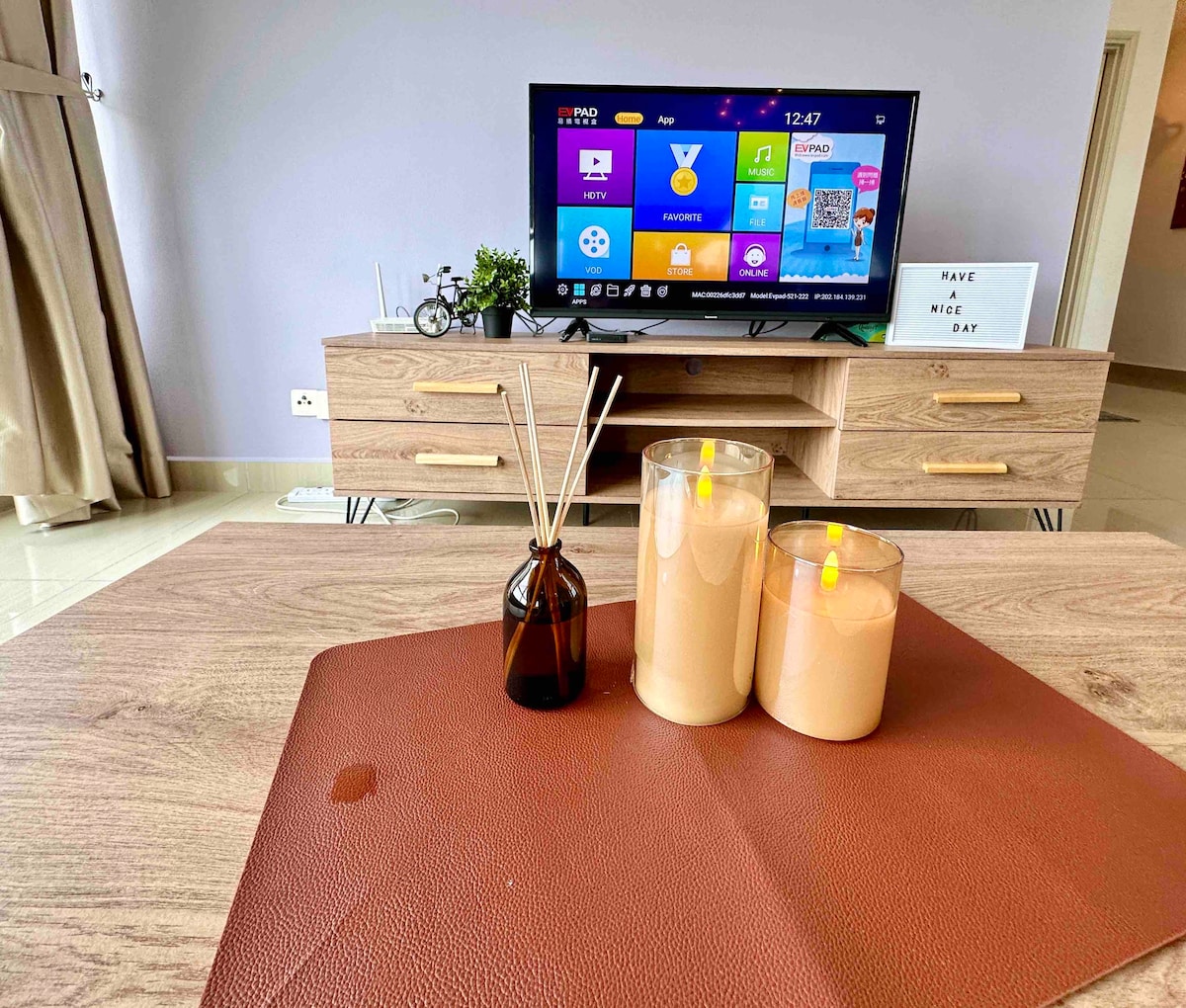In a cozy, well-lit living room, a light tan wooden coffee table takes center stage. Adorned with an orange leather placemat, the table features two white, lit candles—one taller than the other—along with a brown incense jar filled with sticks. A beige bulletin-board-style sign reading "Have a nice day" cheerfully decorates the scene. Flanking the coffee table is a matching TV stand made from similar light tan wood, supporting a sleek flat-screen smart TV. The TV displays a colorful interface with purple and green hues, indicating various app options and the current time. To the right of the TV, a small white sign again offers the warm message "Have a nice day," while to the left, a small plant and a decorative bicycle figurine add a touch of character. The walls of the room are painted a light whitish-blue and are complemented by beige curtains. Natural sunlight floods the room through a nearby window, enhancing the warm and inviting atmosphere.